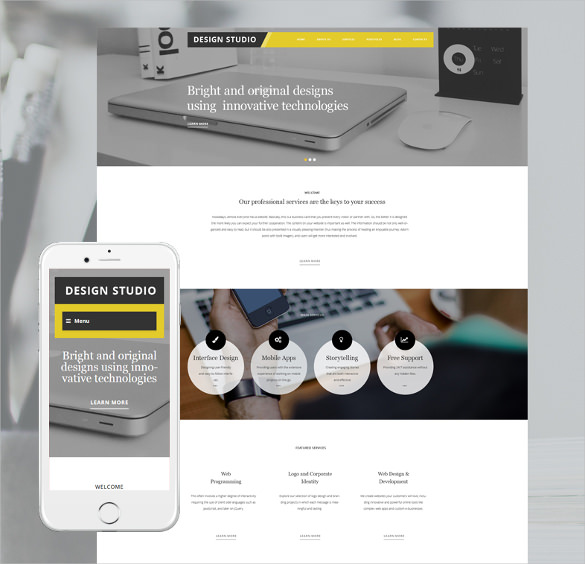The image features a website with a predominantly gray background. At the center, the main section of the page is highlighted in white, creating a stark contrast against the muted backdrop. A prominent top banner showcases the name "Design Studio" in the upper portion of the webpage. Below the banner lies a yellow navigation bar containing six menu items, which are white in color. These menu items are small and somewhat challenging to read due to their size.

The top section of the webpage is dominated by an image of a closed laptop positioned on a gray desk. To the right of the laptop, there is a small rectangular device, while two books are placed on the left. The entire image gives off a black-and-white aesthetic, enhancing the professional and minimalist appearance of the design studio's website.

Additionally, a mobile phone is partially visible at the bottom left corner of the image, emphasizing the website's compatibility with mobile devices. This composition effectively highlights the studio's sleek and modern design approach, suitable for both desktop and mobile viewing.